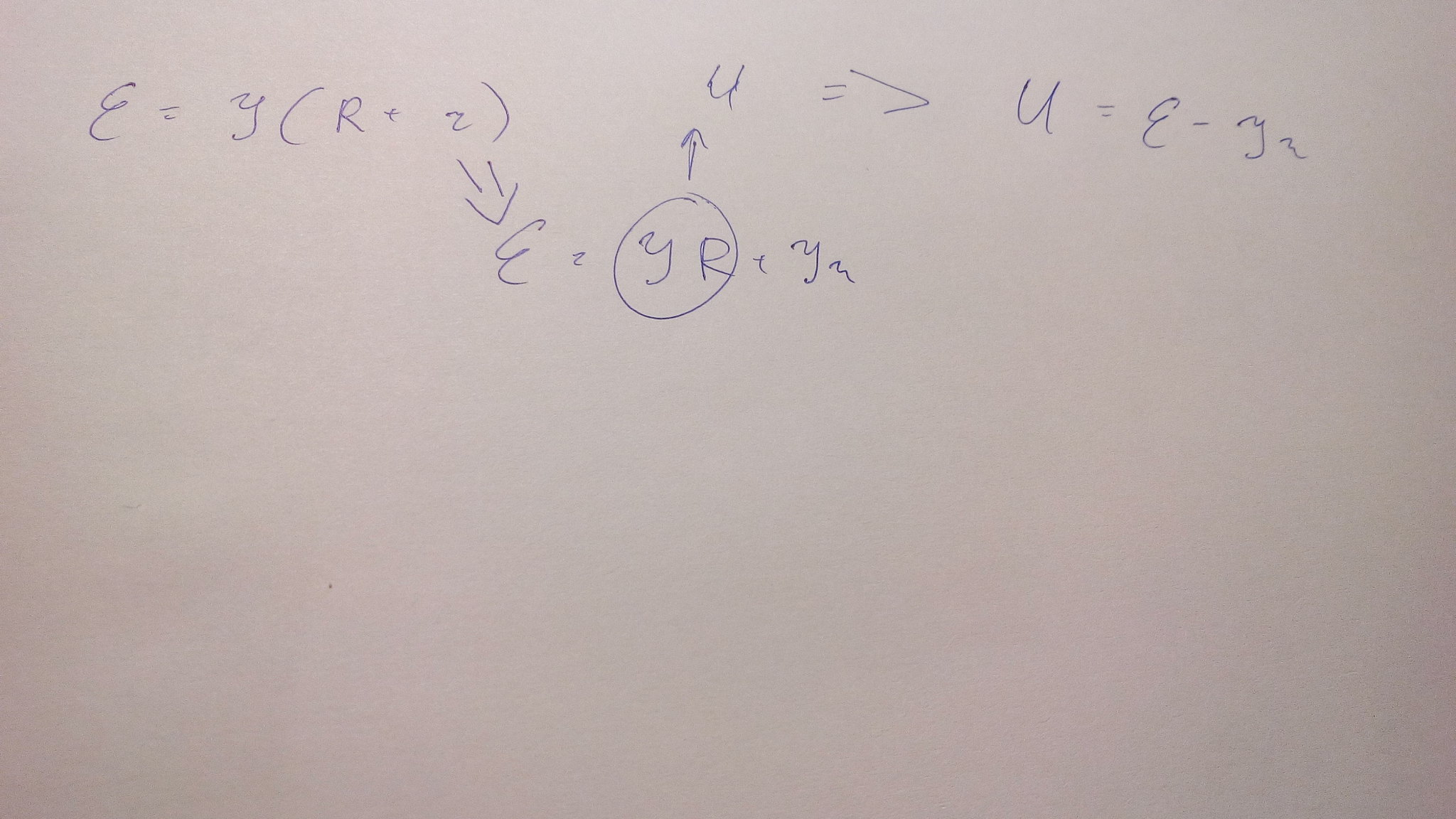A detailed mathematical equation is meticulously handwritten in dry erase marker across the top half of a whiteboard. The equation is divided into two distinct sections, both converging towards a central solution at the bottom. Arrows are drawn, guiding the viewer from the formulas at the top to the final result, which is prominently circled in the middle of the lower half of the whiteboard. Various exponents, values, and equal signs are clearly visible, showcasing the complexity and step-by-step process of solving the formula. The entire scene captures the essence of a focused mathematical problem-solving session.